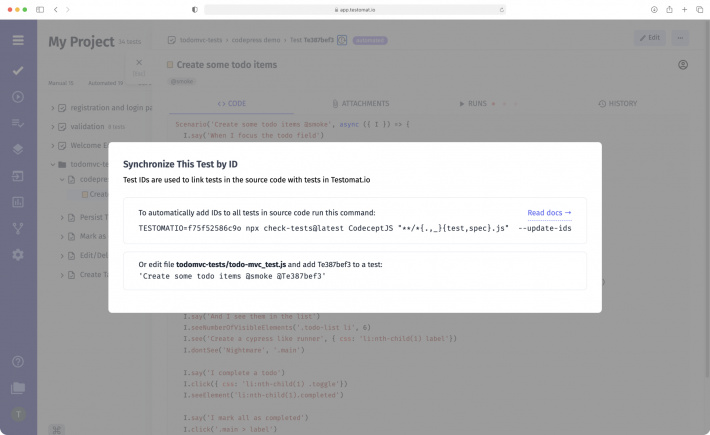A blurry photo captures a detailed view of a web page hosted on some application with a URL that includes "app.something.io." A prominent message overlay slightly obscures the screen, casting a darker shade on the rest of the view. At the top of the page, a header titled "My Project" is visible. A condensed, white-icon menu bar with a purple background is positioned on the left side. Underneath "My Project", there are several tabs labeled "Registration and Login", "Validation", and "Welcome."

The right section of the screen prominently features a text area filled with code. The pop-up message in the foreground has a white background and contains the text "Synchronize this test by ID" in bold. Beneath this, smaller text explains, "Test IDs are used to link tests in the source code with tests in test.mat.io." A subsequent instruction box mentions, "To automatically add IDs to all tests and source code run this command," followed by specific code. Another instructional box at the bottom advises to "edit the file TodoMVCTest.js and add TE387BEF3 to a test."